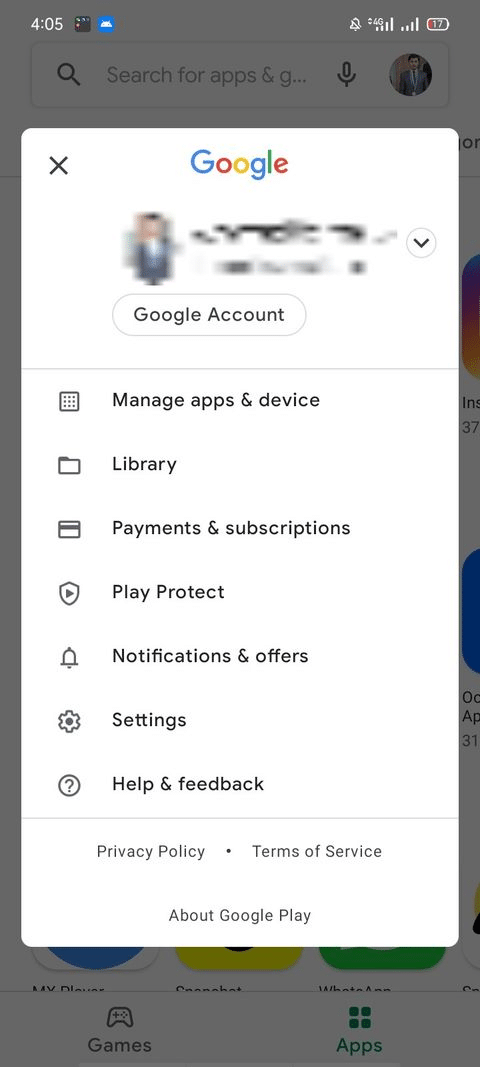The image features a horizontally-oriented phone battery icon in the upper right corner with a small red line, indicating that the battery is nearly depleted. To the left of this, the time is displayed as 4:00. The background is a dark gray, casting significant shadows across the scene. 

Centered in the image is a long rectangular section. At the top left of this section is an 'X' icon, while the word 'Google' appears on the top right. Below this, there is a pixelated area that seems to depict a man wearing a gray jacket with black hair. Further down, the text 'Google Account' is circled.

Continuing downward, there is a calendar icon within a square labeled 'Manage apps and device.' Below this icon and to its right is another square labeled 'Library.' The image then shows a credit card icon within a square with a line at the top, labeled 'Payments and subscriptions.' 

Further down, a shield icon with a small gray line inside is labeled 'Play Protect.' Following this is a section labeled 'Notifications and offers,' which is accompanied by a bell icon. Below this, there is a gear icon next to the word 'Settings.'

Lastly, at the very bottom, there is a circle icon with a question mark inside, beside the text 'Help and feedback.' The footer contains links to the 'Privacy policy,' 'Terms of service,' and information 'About Google Play.'